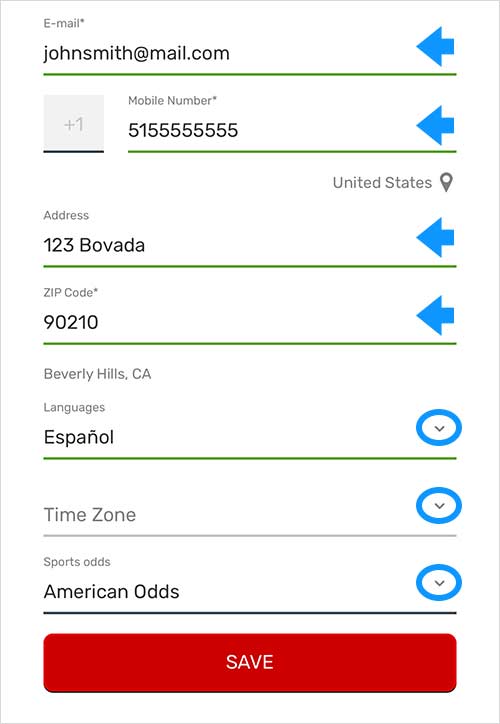This screenshot is of the profile update window within the Bovada online casino platform. The interface is neatly organized, with each section accompanied by visual aids for clarity. At the top, there are four rows with blue arrows pointing to the right, directing attention to each field available for updating.

1. **Email**: The provided email field displays "johnsmith@mail.com".
2. **Mobile Number**: This section includes separate fields for the area code and the mobile number.
3. **Address**: Here, users can input their full address, including a specific section for the zip code.
4. **Languages**: The interface currently shows "Español," indicating the preferred language setting.
5. **Time Zone**: Interestingly, this field shows as “Not Specified.”
6. **Sports Odds**: The system is set to display odds in the "American" format.

For the first four fields, there are blue arrows pointing to them on the right side, guiding users’ eyes to the input areas. For the last three fields—Languages, Time Zone, and Sports Odds—each has a downward arrow encircled in blue, suggesting that these are drop-down menus for further selection options. 

At the bottom of the window, there is a prominently displayed red "Save" button, encouraging users to save their updated profile information.